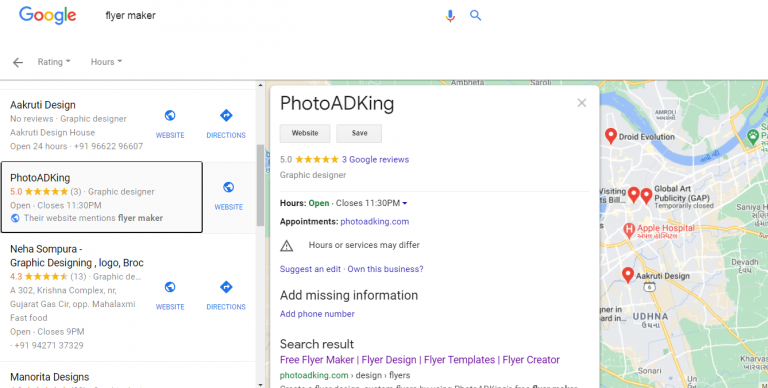A screenshot of a Google search results page is displayed. The familiar colorful Google logo appears at the top left, showcasing a blue "G", a red "O", an orange "O", a blue "G", a green "L", and a red "E". In the search bar, the text "flyer maker" is entered. Adjacent to the search bar, a microphone icon in blue, red, and gold is visible, along with a blue magnifying glass.

Below the search bar, there are navigation options in gray including back arrows, and menu options like "Rating hours." On the left side, search results are listed:

1. **Accurati Design**: A graphic designer with no reviews. Listed as "Accurati Design House", it is open 24 hours and provides a contact phone number.
   
2. **Photo AD Kane**: A graphic designer with three reviews, averaging a 5-star rating. This business is open until 11:30 p.m. The listing notes that their website mentions a flyer maker service.

3. **Naya Sipora**: Described as "Naya Sipora, graphic designing logo Brock," it has 13 reviews and a 4.3-star rating. This business is located at "A302 Krishna Complex NR, Gujarat Gas Circle OPP, Malaxmi," placing it near a fast-food establishment. It is open until 9 p.m., and a phone number is provided.

4. **Mayanora Designs**: This listing is cut off, providing partial information.

To the right, a pop-up window for "Photo AD Kane" details further with a 5.0 rating based on three Google reviews. The business hours are listed, indicating closure at 11:30 p.m. A website link is provided along with options to suggest edits or add missing information like a phone number.

Below the listings, related search results include "free flyer maker," "flyer design," "flyer templates," and "flyer creator."

A map is displayed featuring various landmarks and businesses marked with red location pins. Blue bodies of water and yellow-marked streets are visible. Some highlighted locations include Droid Evolution, Global Art, Publicity Apple Hospital, and Agarwadi Design.

A gray scroll bar is present along the side, suggesting more content below the visible frame.